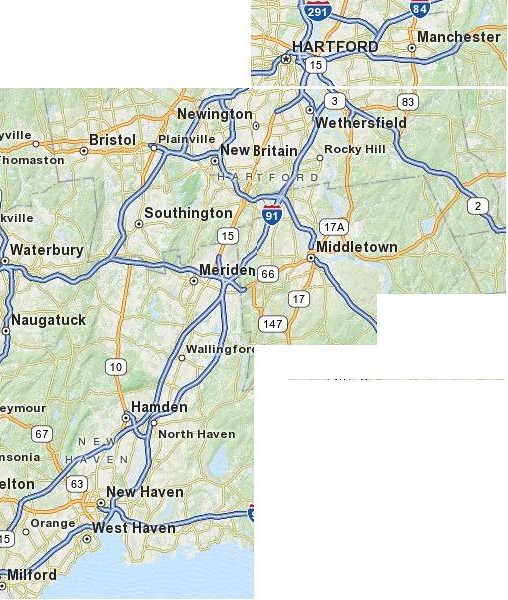This is a low-resolution, vintage-looking screenshot of a roadmap likely taken from a website or digital medium. The map highlights key interstates and local highways with blue and orange lines, respectively, and displays various cities and towns in the Greater New Haven and Hartford area of Connecticut. The cities visible on the map include Hartford, Manchester, Newington, Wethersfield, New Britain, Plainville, Bristol, Southington, Meriden, Middletown, Wallingford, Hamden, North Haven, New Haven, West Haven, Orange, and Milford. The map's design features typical road map elements: green for land, blue for bodies of water, and black for city names. There is noticeable JPEG artifacting, suggesting the image is an old, compressed digital file. The Atlantic Ocean is visible on the bottom left of the map, indicating its coastal geography.